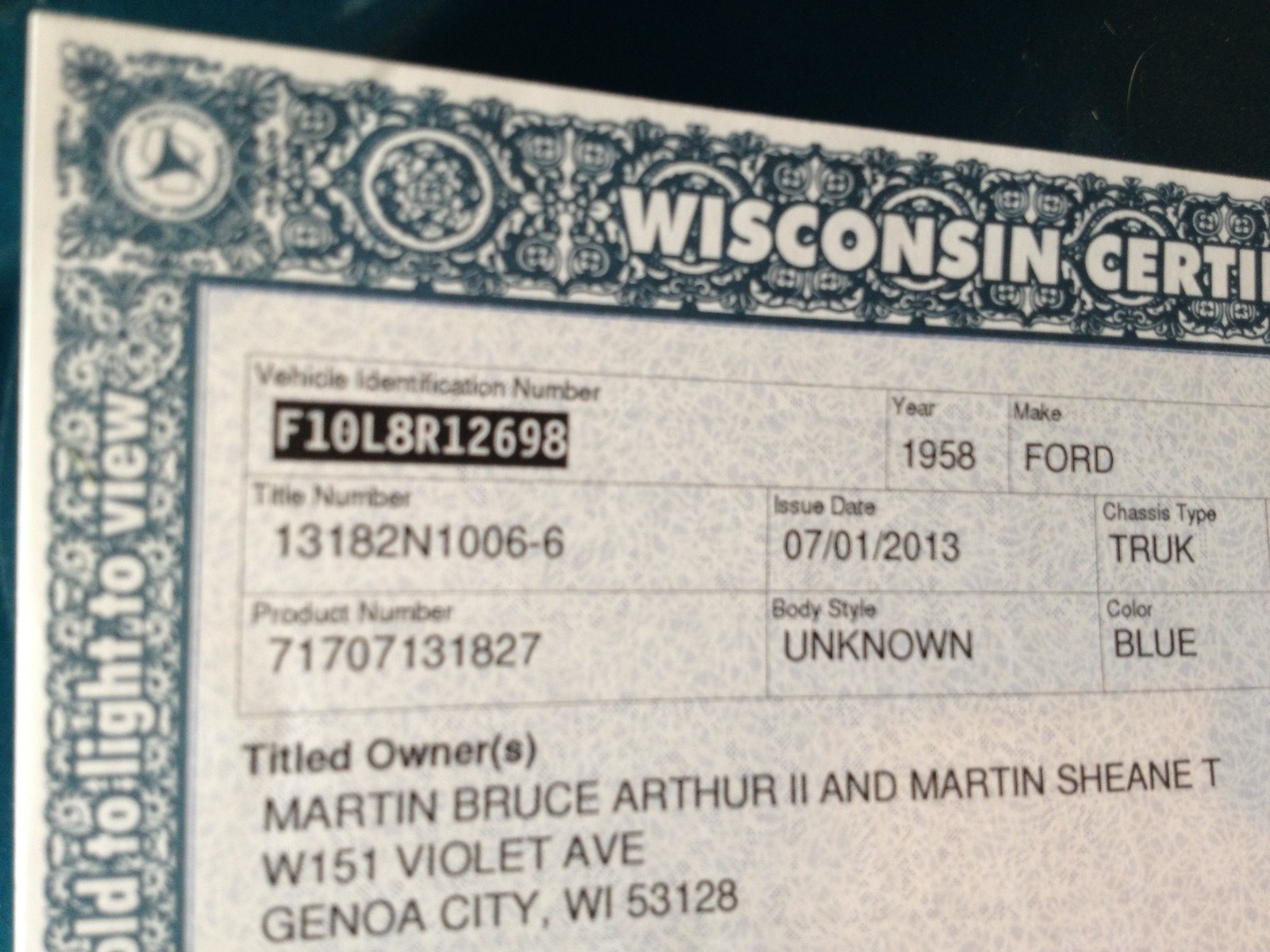The image captures a close-up of an official-looking Wisconsin Vehicle Certificate of Ownership, slightly skewed to the upper left. The document, displaying only parts of its full title, prominently shows "Wisconsin Certificate," C-E-R-T-I partially visible due to the cut-off. On the left side, horizontal text reads "Hold to light to view,” indicating verification features like watermarks. The certificate, bordered with intricate designs and possibly state logos, includes detailed vehicle and ownership information. The vehicle identification number is F10L8R12698, a 1958 Ford truck with title number 13182N1006-6, and an issue date of July 1, 2013. The chassis type is specified as a truck, the product number is 71707131827, body style is unknown, and the color is blue. The titled owners, Martin Bruce Arthur II and Martin Sheen Tee, reside at W151 Violet Avenue, Chenoa City, Wisconsin, 53128. The overall color scheme of the document includes white, dark green, and black.